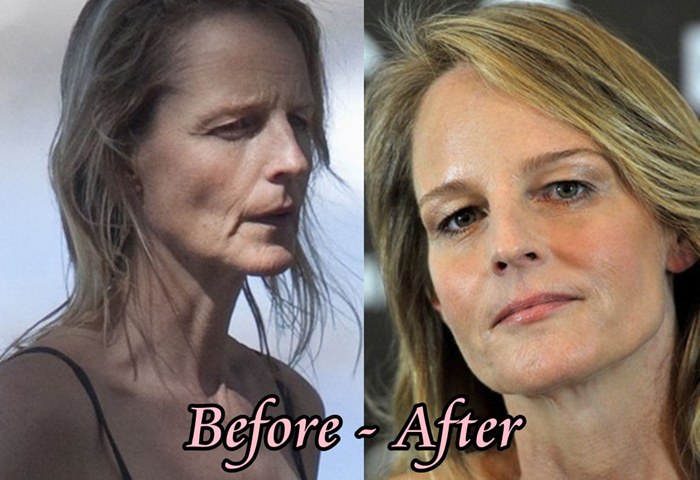The image is a horizontally aligned rectangle divided into two squares. It showcases a 'before and after' comparison of a woman, possibly Helen Hunt, with captions in black-outlined pink, italicized letters stating "Before - After." The 'Before' text is located at the bottom right of the left photo, and 'After' at the bottom right of the right photo, both in a font resembling Times New Roman with an exaggerated tail on the 'F'.

In the 'before' image on the left, the background fades from light gray to pale blue with bright light on the right. The woman appears worn out, too thin, and looking distant and contemplative. Her cheek is sunken with a notable wrinkle from the corner of her mouth, and she’s wearing a strappy top with bare shoulders. Her blonde hair, slightly past chin length, looks pushed back near her ears, creating a somewhat messy impression, as if damp around the temples.

In the 'after' image on the right, the background is black adorned with white, pill-shaped designs. The woman looks healthier, with a more filled-out face and makeup on her cheeks. Her hair appears fuller and styled, giving a fresh, blown-dry look. She is making direct eye contact with the camera, projecting confidence and beauty. The transformation highlights her improved appearance and overall well-being.